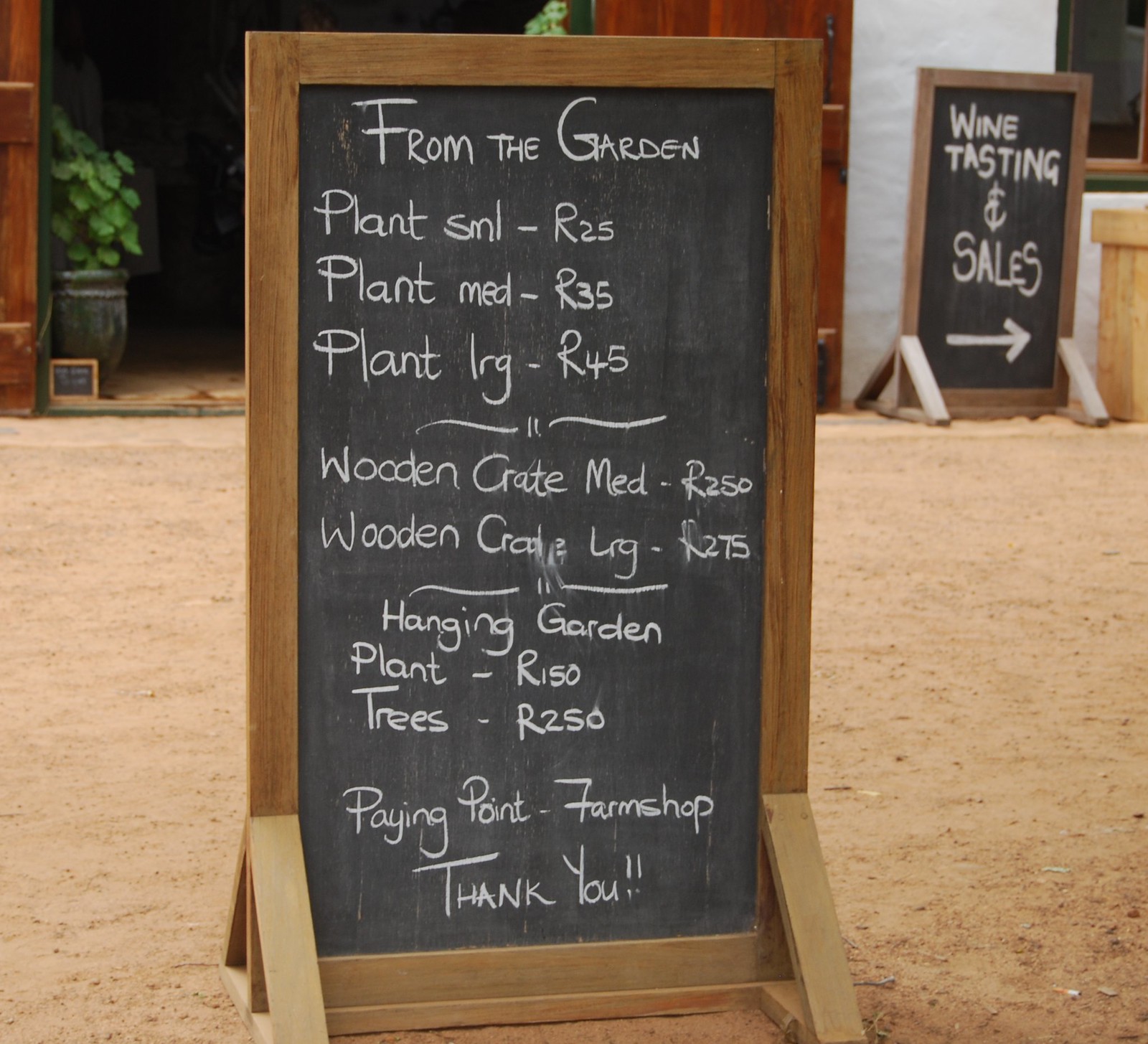This daytime photograph captures a rustic wooden sign constructed from a combination of wood and a central chalkboard. Written in white chalk, the sign details various garden products and their prices, starting with "From the Garden." Below this heading, the sign lists: "Plant SML - R25," "Plant MED - R35," and "Plant LRG - R45," featuring a decorative swirling design below these listings. Further down are prices for crates: "Wooden crate MED - R250" and "Wooden crate LRG - R275," followed by another swirling design. Additionally listed are: "Hanging garden plant - R150" and "Trees - R250," culminating in "Paying point - Farm Shop" with a pair of exclamation points. The sign is set against a backdrop of golden dirt, and scattered around it are a few cigarette butts. In the top right corner of the image, another similar sign can be seen bearing the message "Wine Tasting and Sales" with an arrow pointing to the right. The overall scene suggests an outdoor setting at a farm or garden shop.